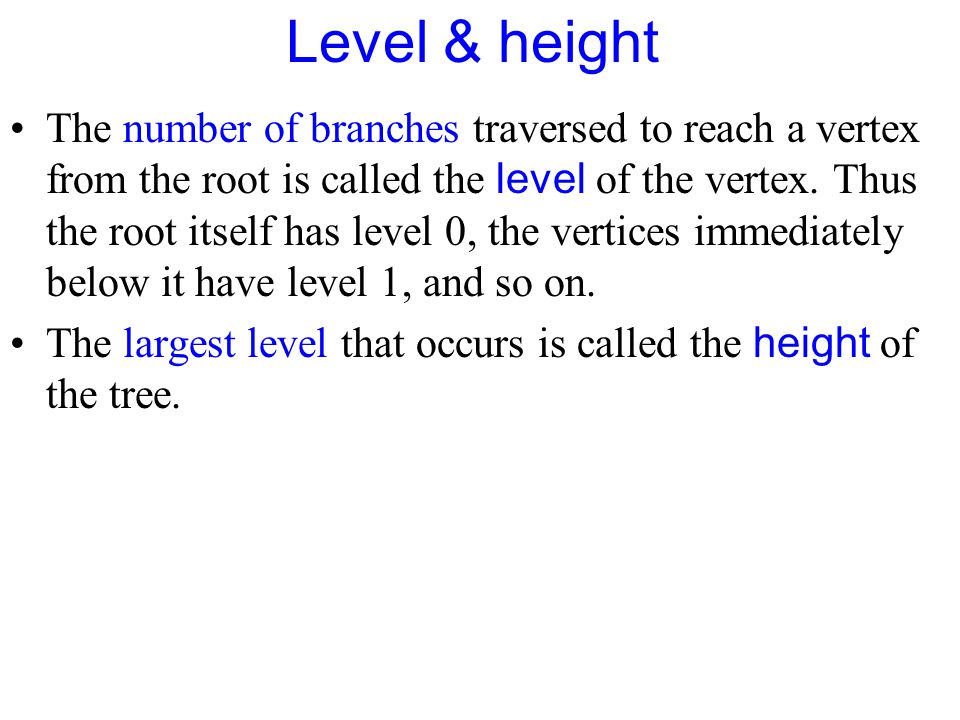The image displays text-only content on a plain white background, resembling a slide from an online course. Centered at the top, there's a title in blue text reading "Level & Height." Below the title are two bullet points, each introduced by a black circular bullet on the left. The first bullet point explains, "The number of branches traversed to reach a vertex from the root is called the level of the vertex. Thus, the root itself has level 0. The vertices immediately below it have level 1, and so on." In this bullet point, the phrases "number of branches" and "level" are highlighted in blue. The second bullet point reads, "The largest level that occurs is called the height of the tree," with "largest level" and "height" also highlighted in blue. The text alternates between blue for key terms and black for the rest of the description, providing a clear and structured explanation of tree data structure terminology.